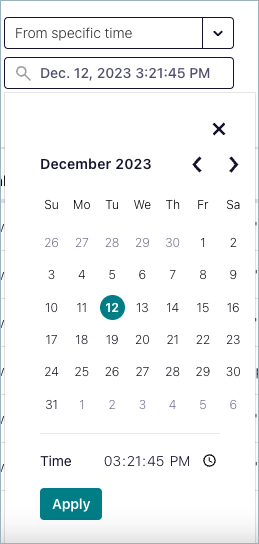The image depicts a straightforward digital calendar interface for December 2023. The layout is minimalistic with a predominantly white background. The focus is on an appointment scheduled for December 12th, clearly indicated by an indigo-colored circle around the date. Below the calendar grid, there is a detailed section specifying the time of the appointment set for 3:21:45 PM. Adjacent to this time setting, there is a functional button labeled "Apply." At the top of the page, a search bar displays the same date and time—December 12th, 2023, at 3:21:45 PM—suggesting a streamlined way to find and manage specific appointments. An option to select a specific time range is also available, highlighted by an arrow icon on the right side of the search bar. The text and numbers on the calendar are in black, providing a clear contrast against the white background for easy readability.